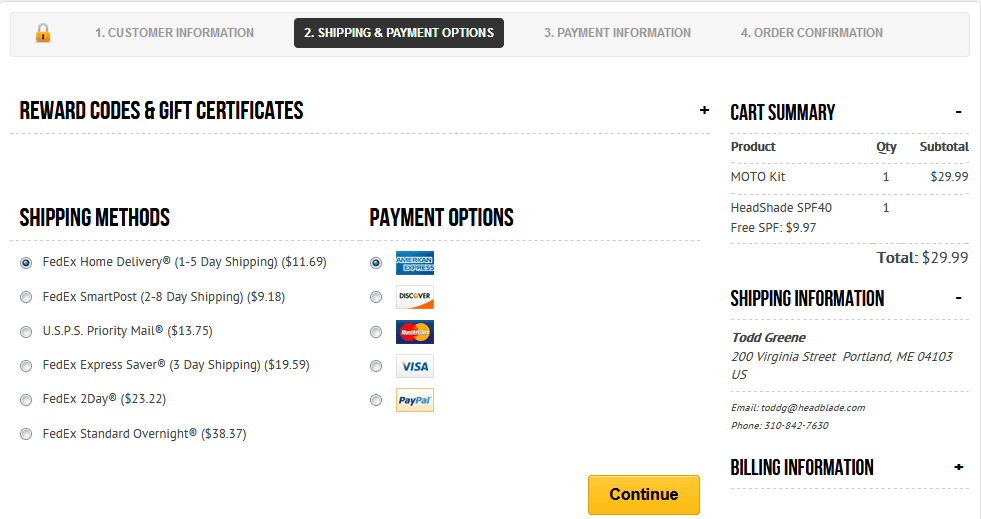This image depicts a payment screen on an e-commerce website with a design similar to Amazon's. The interface is predominantly white, featuring a yellow "Continue" button at the bottom. In the top left corner, "Customer Information" is labeled next to a lock icon, symbolizing security. Adjacent to it, the navigation bar highlights "Shipping and Payment Options," and subsequent tabs include "Payment Information" and "Order Confirmation."

Below the navigation bar, there is larger, bold, all-caps text reading "REWARD CODES AND GIFT RECEIPTS," accompanied by a plus symbol to its right. Below this section, another text block reads "Card Summary," marked with a minus symbol indicating collapsibility. Further down, there are details for "Product Quantity" and "Subtotal" displayed in slightly smaller bold black text.

In the shipping information section, it lists an address formatted neatly beneath the product summary. Six shipping options are presented vertically to the left of the reward codes section: FedEx, Smart Post, USPS or Email, FedEx 2 Day, and Send It Overnight. These options provide users various choices for delivery methods. The overall layout is clear and organized, ensuring a user-friendly experience.